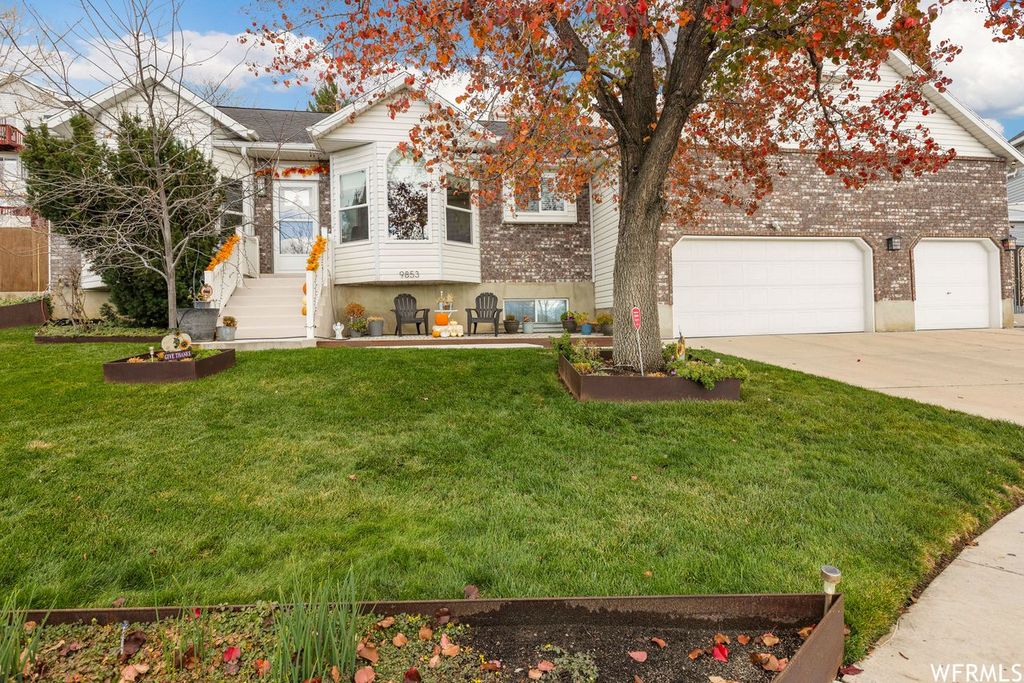The image shows a large, suburban, one-story home with a mix of brown and white brick exterior accented by white wooden siding and a grey roof. Prominent in the front yard is a spacious driveway leading to a three-car garage, featuring two white garage doors, one large for two cars and another smaller for a single car. The front of the house includes bay windows and about six or seven steps leading up to a white front door, which is complemented by a screen door with glass panels. Decorated for fall, the yard features several pumpkins lining the staircase and walkway, indicative of Halloween with additional decorations scattered around. The neat, recently mowed lawn appears slightly lumpy but well-maintained. The front yard boasts a large tree with vibrant red leaves, alongside another tree that is completely bare, further emphasizing the autumn season. On this bright, sunny day without overcast skies, the house sits elevated on a three-foot base, presenting a picturesque and welcoming environment true to a suburban setting.